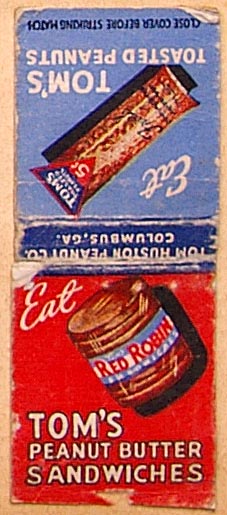This image features the cover of a vintage matchbook from the Tom Houston Peanut Company, located in Columbus, Georgia. The design is divided into two distinct color sections: blue on the top half and red on the bottom half.

**Top Half:**
- At the bottom of the top half (considered upside down in the image), there is a prominent dark blue line with the text “Tom Houston Peanut Company, Columbus, Georgia.”
- Above this line, the background transitions to light blue, and in white cursive text, angled slightly, it says "Eat Tom’s Peanuts."
- Diagonally from the upper right corner to the lower left corner, there is an illustration of a package of Tom's Peanuts priced at five cents, featuring additional blue writing.
- Below the illustration, in all capital letters and white text, it reads "Tom's Toasted Peanuts."

**Bottom Half:**
- The background is entirely red with some areas showing blue peeling at the top.
- In the center, in bold white text, it says "Eat Tom's Peanut Butter Sandwiches."
- To the right, there is an image of a peanut butter jar labeled "Red Robin" with red letters on a blue label. The jar is oriented towards the upper left corner with its bottom facing the lower right corner.
- At the very bottom, the safety warning "Close Cover Before Striking Matches" is printed.

**Condition:**
- The matchbook has visible wear and tear, with paper separation at the upper right corner and worn edges showing "bumps and bruises."

The entire image is set against a taupe-colored piece of paper, adding to its vintage appearance.